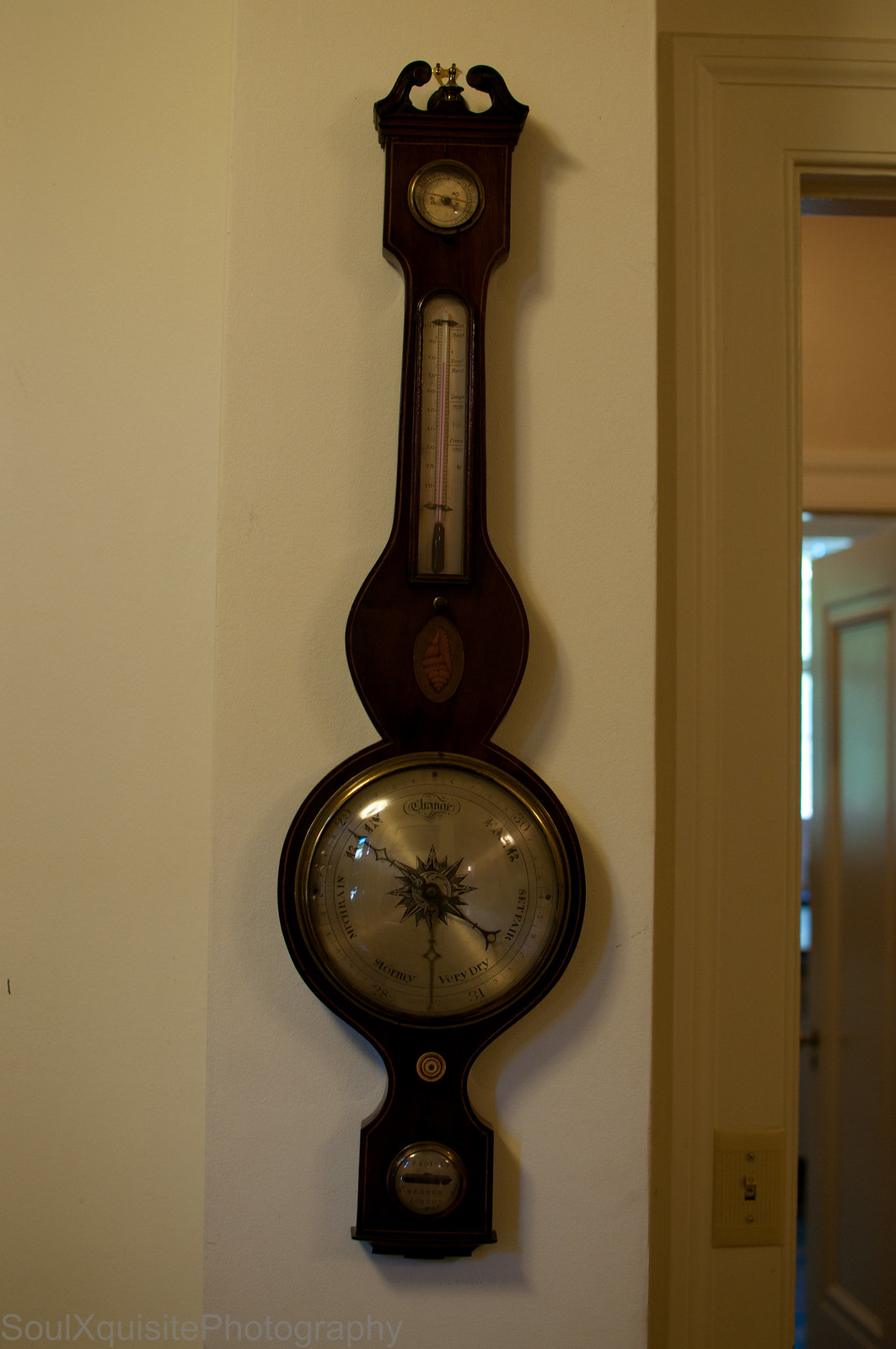This color photograph depicts a vintage wooden barometer mounted on a beige wall, positioned next to a golden ochre door frame with a light switch. The barometer showcases an early American design, with an elongated form that tapers into a neck shape at the top. This neck features a thermometer, though the details are too distant to discern clearly. Below the thermometer, there's a gold-faced circular dial, presumably the barometer, encased in glass with at least one visible arm, though additional details are indiscernible. At the very top of the barometer is a small circular dial, whose specifics are not clear due to the distance. The overall structure transitions from a narrow neck to a broader circle, finishing with a square base. A watermark, "Sol Exquisite Photography," is visible at the bottom of the image.